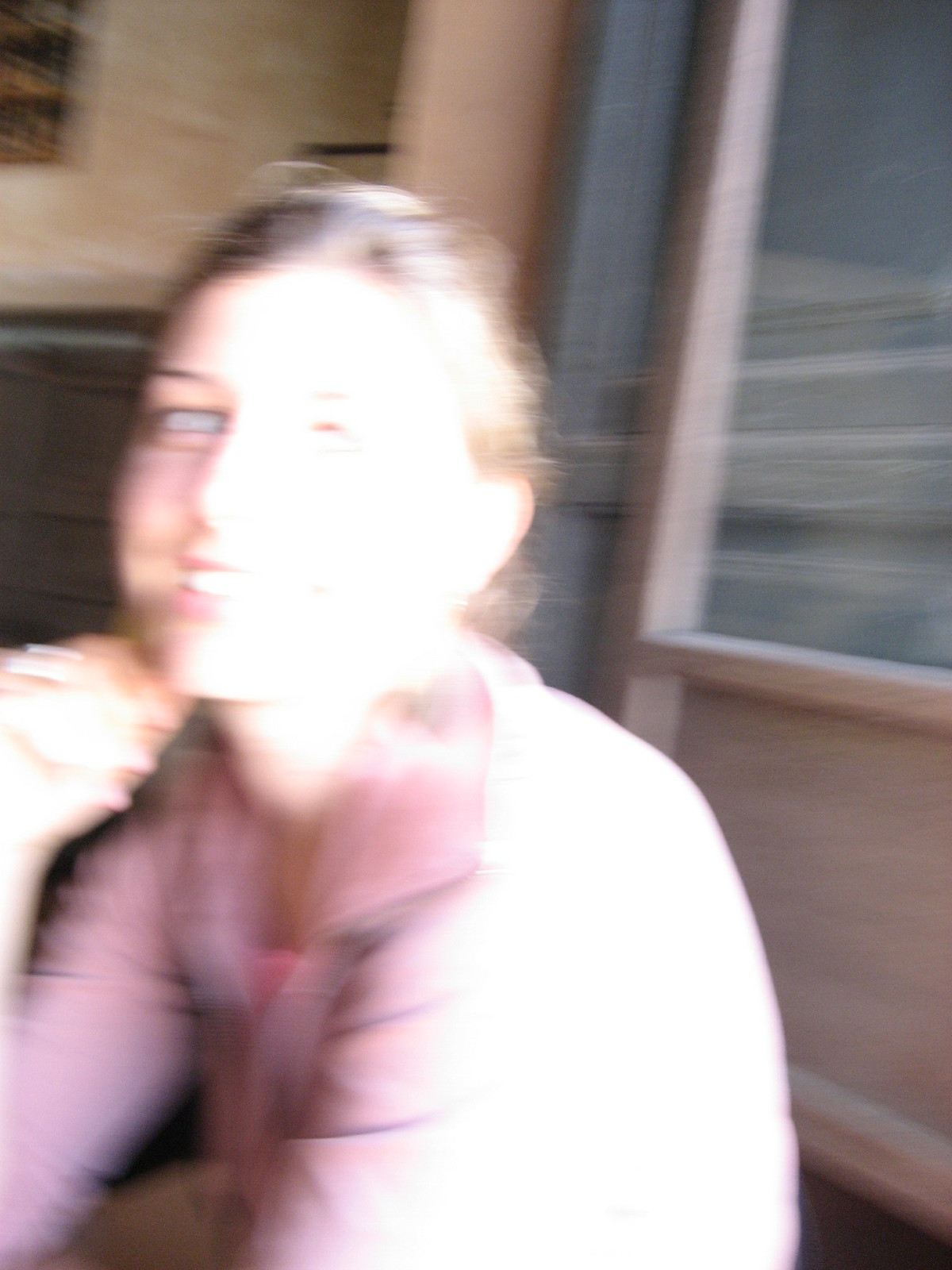This photograph captures a blurred image of what appears to be a woman, suggesting the photographer was in motion while taking it. The main subject, likely stationary, is posing with her chin resting on her left hand. The woman, who has dark brown hair possibly tied back into a ponytail, is featured prominently on the left side of the image. Visible facial features include her eyes, eyebrows, and a subtle smile. The woman is dressed in a long-sleeved pink hoodie layered over a pink shirt.

The background hints at an indoor setting, potentially inside a restaurant or a train compartment. The walls are predominantly light rust-colored with dark gray or green borders extending midway down, creating a distinct two-tone effect. Additionally, there is a door or window in the background, painted a light brown shade, contributing to the warm, enclosed ambiance of the scene.